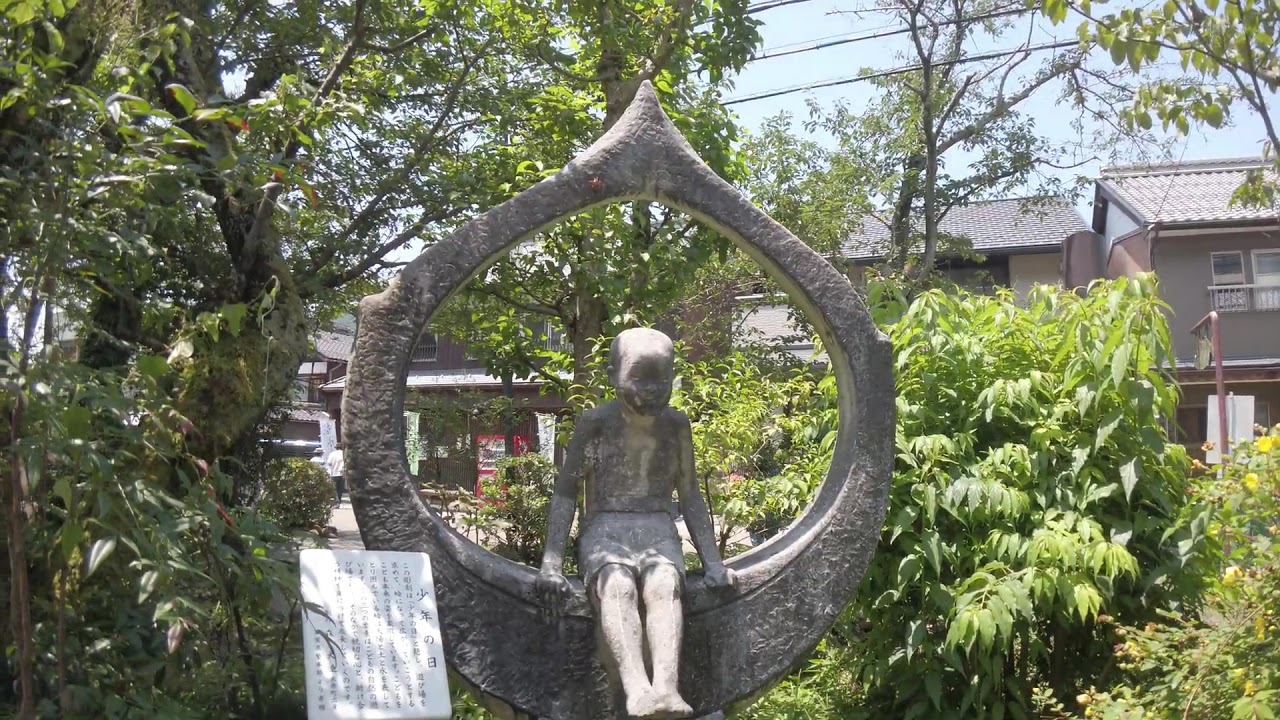This photograph captures a detailed scene of a stone sculpture situated in a lush garden flanked by trees. The centerpiece is an open circular sculpture with a pointed top, featuring a stone statue of a small child, apparently a boy, seated inside. The child's hands are placed on the edge of the circle, and his legs dangle slightly outward, clad in shorts that expose his knees and toes. 

To the left of the sculpture, there's a white plaque inscribed with black Asian—likely Japanese—characters, and another similar plaque can be seen to the right. The background reveals a two-story dwelling extending across the entire width of the photograph, partially obscured by the trees. Hints of additional buildings, electrical lines, and a blue sky add depth to the backdrop. The composition is enriched with verdant bushes and branches, creating a serene yet intricate setting.